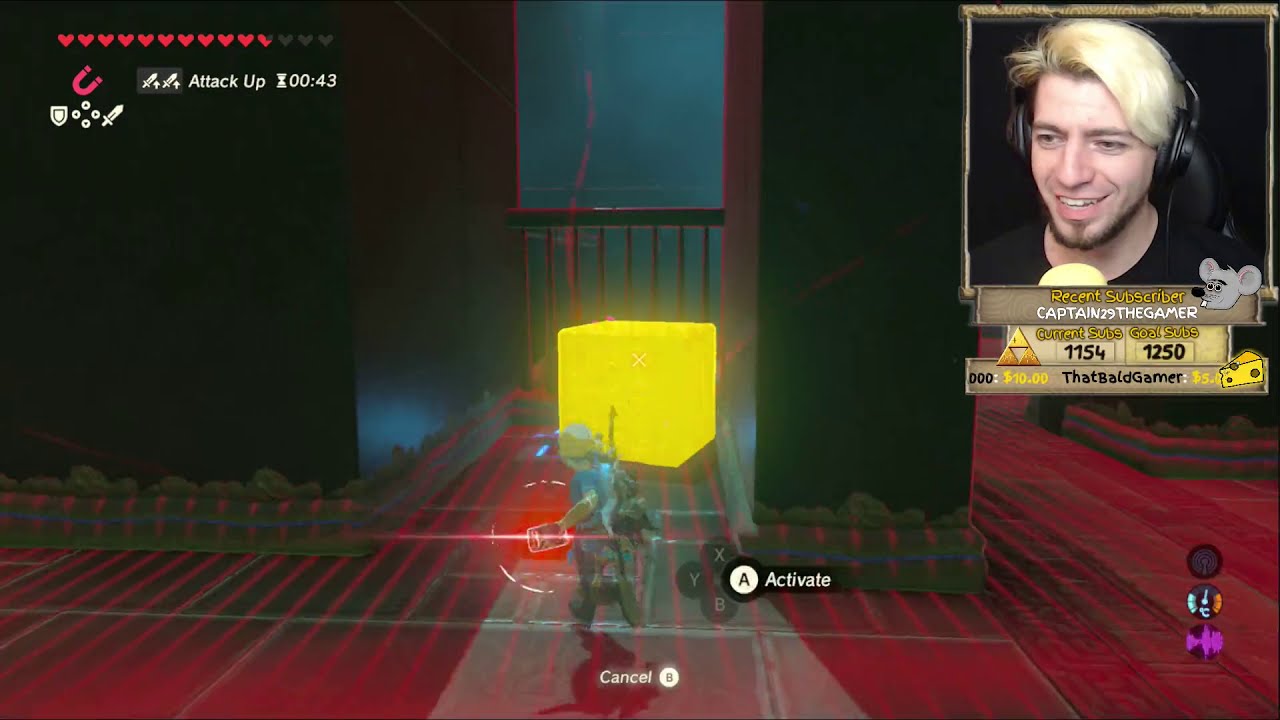A detailed screenshot from a video game depicts a character, possibly a soldier, maneuvering to the left with a bright yellow cube behind them and a dark maroon barrier in the background. The character, though somewhat foggy, appears to be holding a weapon and possibly drinking a red juice, suggesting a power-up. The floor features a pattern of red and gray rectangles. In the upper left corner, a display shows "Attack Up" with a timer at 00:43, accompanied by a red horseshoe magnet, and a line of hearts where three and a half are unfilled. There are additional icons, likely indicating stats or items, including a shield and a sword.

In the upper right corner, there's a webcam feed of a man with blonde hair parted to the left, a brown beard, black microphones, and a smile. His name, "Captain29thegamer," is shown with "Recent Subscriber" highlighted in yellow. Below his image are his current score of 1154 and a subscription goal of 1250. Adjacent are icons and numbers, including a $10 and $5 marker flanked by a piece of cheese, possibly donation alerts. The text "That Bald Gamer" is visible near these icons. The bottom of the screen displays the word "cancel," with "activate" just behind the character, surrounded by the letters A, X, Y, and B, indicating game controls.